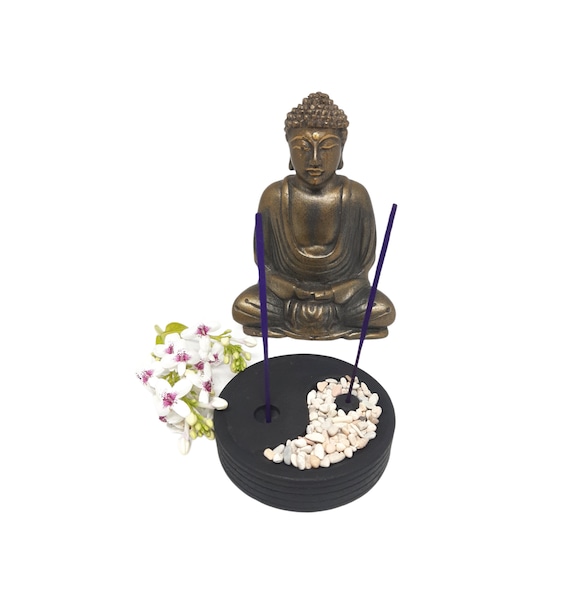This aerial photograph, set against a completely white background, captures a serene altar scene from a Southeast Asian temple. Dominating the upper part of the image is a brass-colored statue of a Buddha-like deity, sitting calmly in a lotus pose with crossed legs, closed eyes, and a slightly pursed mouth. The deity wears a traditional honeycomb-patterned hat and an intricately creased fabric garment. In the foreground, we see a round black incense holder with two stands, each holding a burning stick of bluish-purple incense. Small white and gray pebbles are artfully arranged around the right hole to form the yin sign. To the upper left of the incense holder lies a group of delicate white star orchids with vibrant purple throats and green leaves, adding a touch of natural elegance to the spiritual scene.